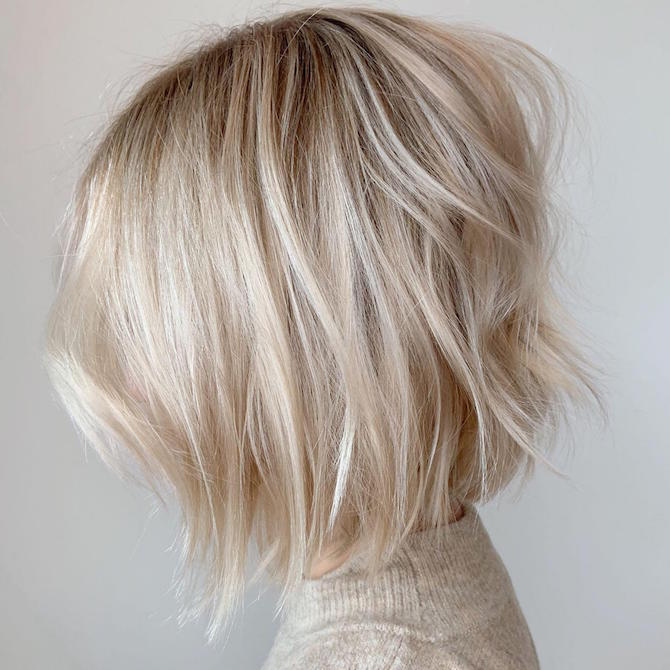The photograph captures a side view of a woman’s recently cut, layered hair. Her bleach blonde hair, with slightly browned roots, falls to just above her shoulders. The style appears somewhat disheveled, demanding a comb. She’s donned a soft, light-colored turtleneck sweater that contrasts subtly against her pale hair—a detail mirrored in the background, which is a plain white wall. The composition of the image focuses solely on her head, with her face turned to the left, resulting in her face being out of the frame, giving prominence to her hairstyle. The minimalist, indoor setting emphasizes the freshly styled hair, suggesting she’s showcasing the new haircut.